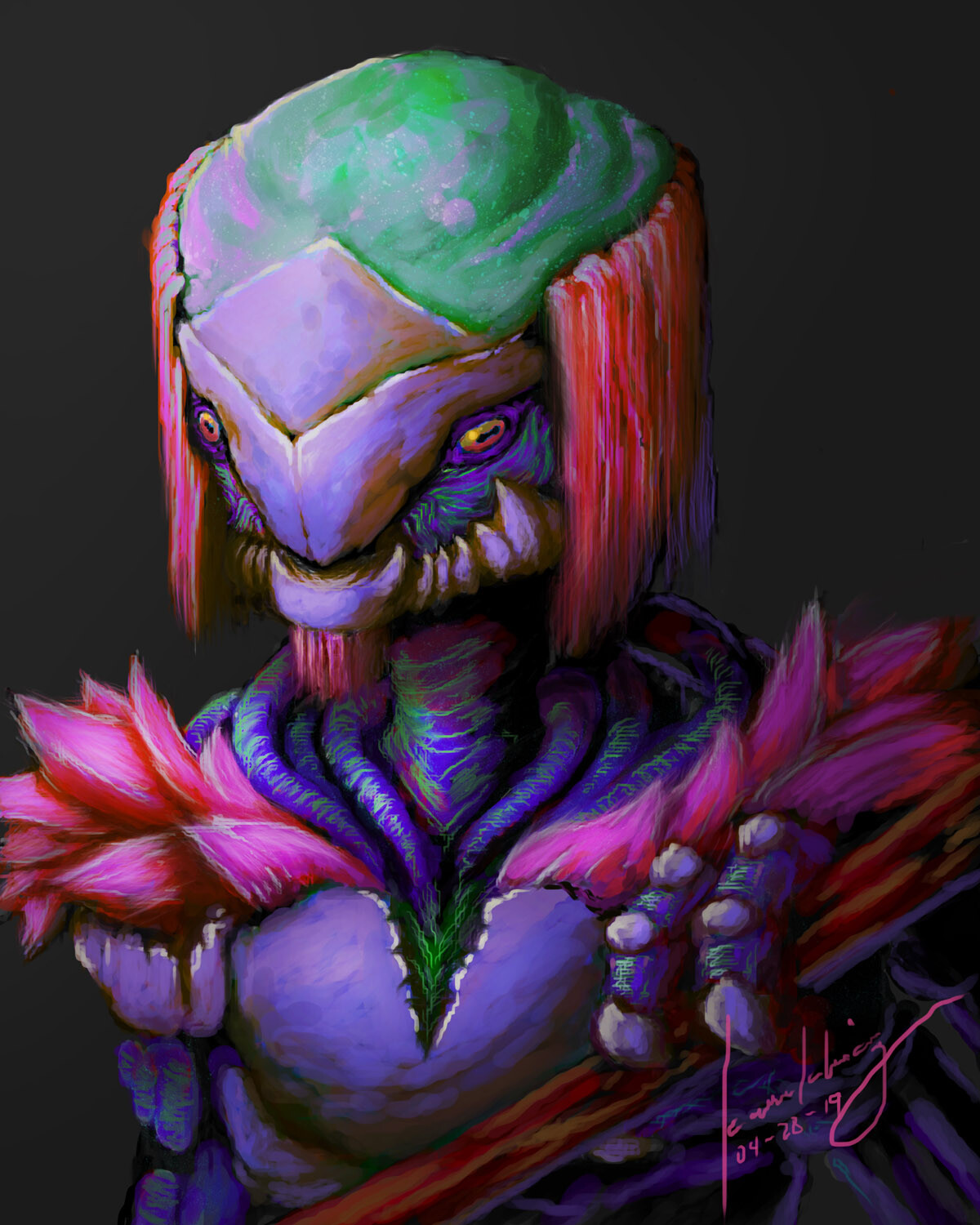This detailed painting portrays an alien figure set against a black background, vividly brought to life through a mix of bright colors, predominantly purples, greens, pinks, and hints of oranges. The alien's head is striking, characterized by a large green scalp with a tarantula-like texture and long orangish-pink hair cascading from the sides. The creature's eyes are a mesmerizing golden yellow with black retinas. Its purplish-hued skin contrasts beautifully with its elaborate attire—a sleeveless top adorned with pink feathers extending from its shoulders, which resemble scaled shoulder pads. The alien clutches a thin wooden stick, adding a sense of warrior-like presence to the figure. The artist's signature, dated 04-28-19, is inscribed in pink in the bottom right corner of the painting, marking it as a distinctive and imaginative artwork.